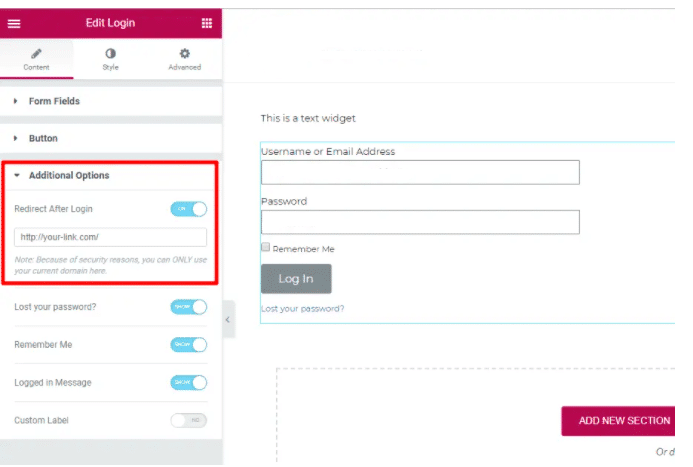The image displays a user interface for a login form on a website. The form includes several elements and options for users to interact with. At the top, there is a text widget prompting the user to enter either a username or an email address, followed by a text field for input. Below this, there is another text field for the user to enter their password. Adjacent to the password field, there is a 'Remember Me' checkbox that users can select if they want the site to remember their login information for future visits.

The form also includes a 'Login' button for users to submit their information and gain access to the site. Below the login button, there is a 'Lost your password?' link for users who need to reset their passwords. Additionally, there is an 'Add new section' option, outlined by a gray dotted line, which might be for further customization or administrative purposes.

A blue border highlights the active form fields, including the username/email input, password input, 'Remember Me' checkbox, 'Login' button, and 'Lost your password?' link, indicating where users can interact with the form. A separate text section at the bottom indicates advanced options like editing the login content style, form fields button, redirecting after login, and additional options like custom labels and logged in messages.